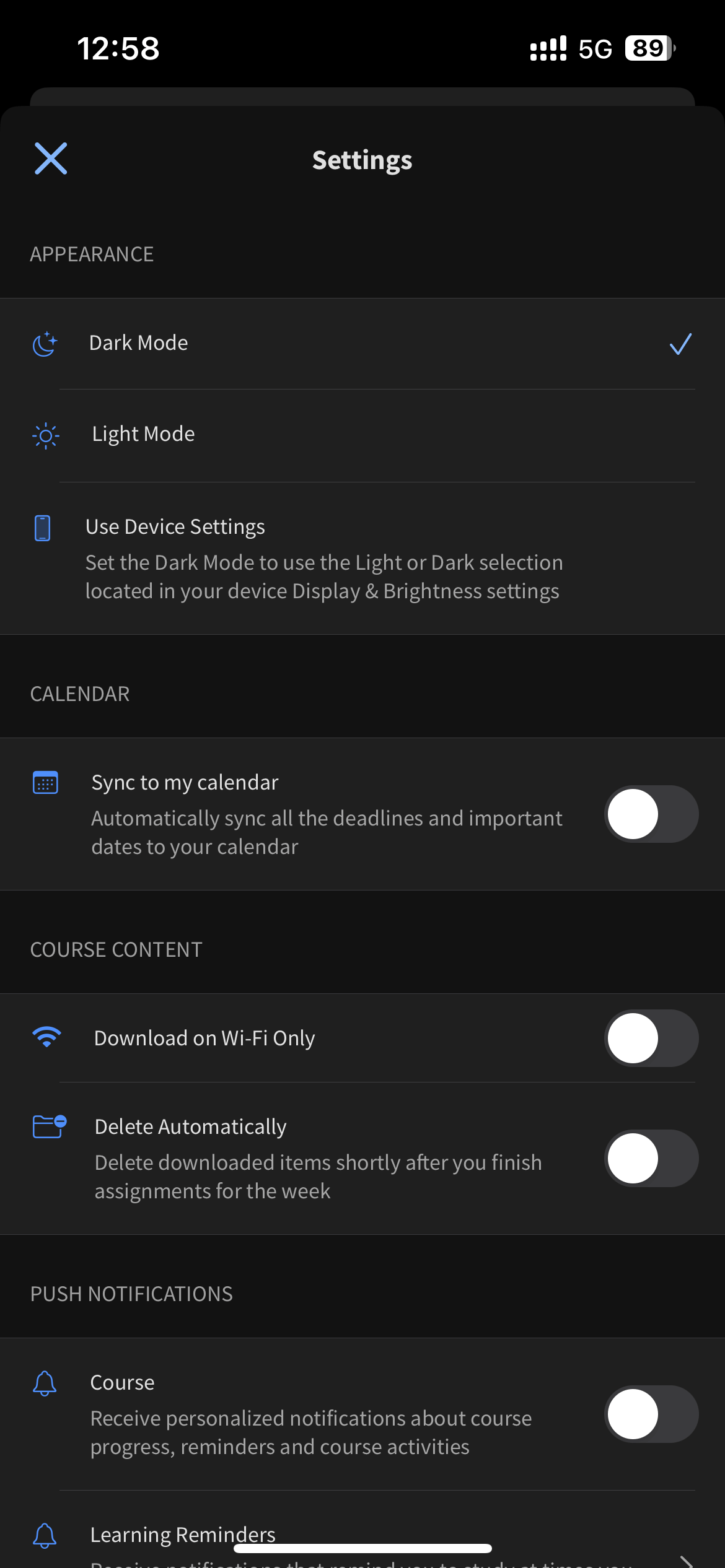A screenshot from an Android phone captures a settings menu with a predominantly blue background. The status bar at the top includes the time (12:58), full signal strength (five out of five bars), a 5G connection indicator, and a battery level at 89%. In the top middle of the screen, the word "Settings" is prominently displayed, while a blue "X" is situated on the upper left side.

Below this header, the "Appearance" section is visible with the following options:
- Dark Mode: checked
- Light Mode: not checked
- Use Device Settings: with a description that reads, "Set the dark mode to use the light or dark selection located in your device display and brightness settings."

Further down, the "Calendar" section is shown with the option to "Sync to my calendar," which states, "Automatically sync all the deadlines and important dates to your calendar." This option is toggled off.

Next, under the "Course Content" section, two additional toggles are seen:
- Download on Wi-Fi only: toggled off
- Delete automatically: toggled off

Finally, the "Push Notifications" section is visible, displaying the options for "Course and learning reminders," which are also toggled off.